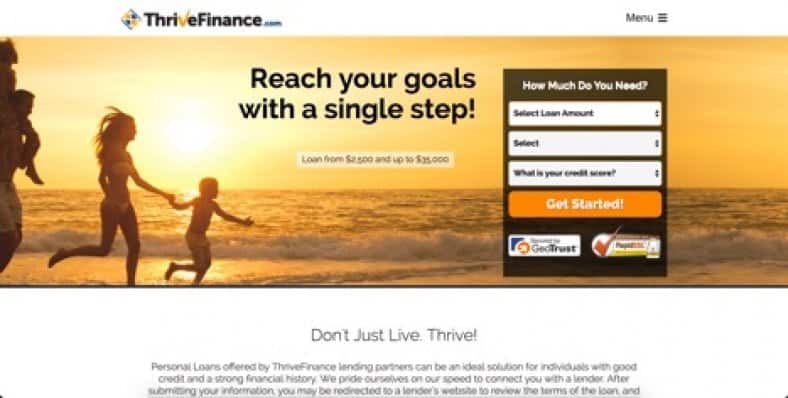Here's a cleaned-up and detailed caption for the image:

---

The homepage of Thrive Finance features a clean and modern layout aimed at providing easy access to financial services. At the very top, a white navigation bar contains a 'Menu' button represented by three horizontal lines on the right side. To the left, the Thrive Finance logo is prominently displayed; the 'V' in the word 'Thrive' is highlighted in yellow, while the rest of the text is in bold black, and 'dot com' is in a small blue font. 

Beneath the navigation bar, a picturesque background of a golden sunset by the beach sets a serene and hopeful tone. The image captures a family enjoying the beach — a man with a child on his shoulders, a woman running in a bikini, and another child playing, symbolizing freedom and joy. Central to this image is the motivational message in bold black text: "Reach Your Goals with a Single Step".

Further down, within a light yellow box, there is a brief promotional note in gray text mentioning loan offerings ranging from $2,500 up to $25,000. To the right, a functional black box invites users to engage with the loan application process. At the top, in white text, it asks "How Much Do You Need?" followed by a white box for selecting the loan amount with black writing. Below that, users can select their credit score from a dropdown menu. The call-to-action button in an orange box with off-white text reads "Get Started". 

At the bottom, two small verification icons add a sense of security; the left one likely says "GeoTrust," and the right one features a red check mark, though its label is not fully visible. The footer reminds users, "Don't Just Live, Thrive," accompanied by additional information about personal loans in gray text.

---

This comprehensive caption captures the essence and details of the webpage's design and message, providing a clearer understanding of its visual and functional elements.